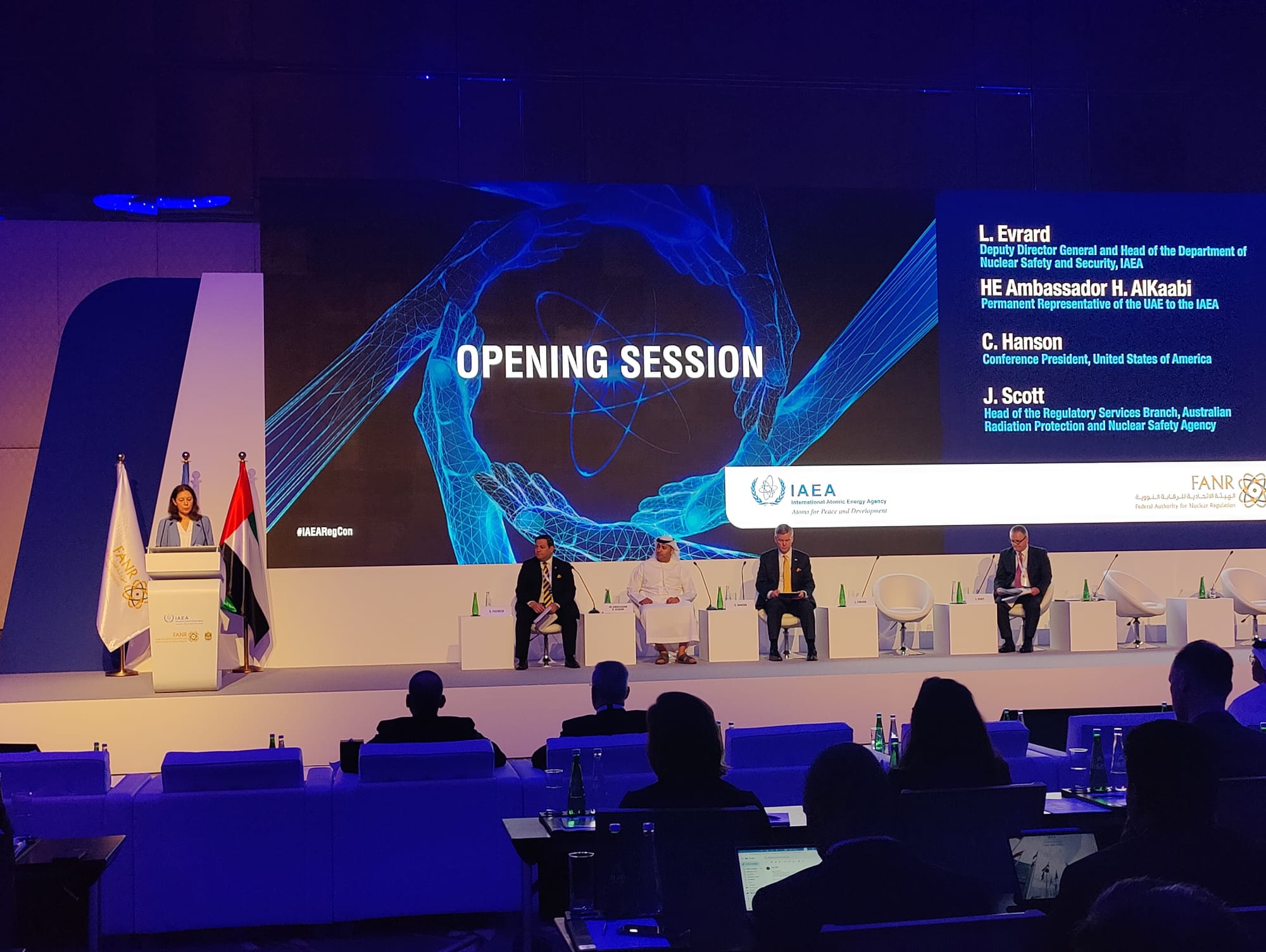The photograph captures a significant event, likely a seminar or press conference, organized by the IAEA (International Atomic Energy Agency). The focal point is a stage where four individuals are seated, including three men in suits and one wearing Middle Eastern attire. A woman, dressed in a blue suit, stands at a podium to the left side of the stage, with a backdrop of numerous flags behind her. Above the seated people, a large screen prominently displays a series of blue hand graphics curling into a circular shape, with the text "Opening Session" overlapping the graphic. The names and titles of the distinguished speakers include El-Evard, the Deputy Director General and Head of the Department of Nuclear Safety and Security at IAEA; H. Al-Khabi, the Permanent Representative of the UAE to the IAEA; C. Hansen, the Conference President from the United States of America; and J. Scott, the Head of the Regulatory Services Branch at the Australian Radiation Protection and Nuclear Safety Agency. The audience, visible through the first few rows, is formally dressed, with attendees donning suits and dresses, and having water bottles at their seats, indicating a formal and well-organized event.